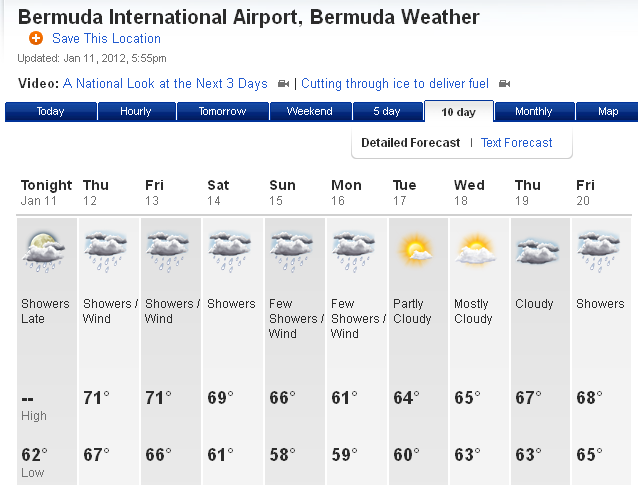The image is a horizontal screenshot depicting a detailed weather map for Bermuda International Airport. In the upper left corner, it indicates "Bermuda International Airport, Bermuda Weather," with a plus icon and the option to "Save this Location" just beneath it. This data was last updated on January 11, 2012, at 5:55 PM.

Directly below, there is a section titled "Video" featuring two blue hyperlinks: "A National Look at the Three Days" and "Cutting Through Ice to Deliver Fuel." The bottom portion of the image displays a toolbar with dark blue gradient buttons that allow users to scroll through different forecast options. These options are labeled as "Today," "Hourly," "Tomorrow," "Weekend," "Five Day," "Ten Day," "Monthly," and "Map," with "Ten Day" being the selected option.

Under the toolbar, there are two choices for viewing the forecast: "Detailed Forecast" or "Text Forecast." The forecast itself reveals icons representing various weather conditions such as rain clouds and sun. The leftmost column is labeled "Tonight," indicating "Showers Late" with an unmarked high and a low of 62°F.

The weather forecast spans from January 12th (Wednesday) to January 20th (Friday), using alternating light gray and medium gray columns for each day. The highest temperature for the week is forecasted to be 71°F, while the lowest temperature is expected to be 58°F on Sunday.